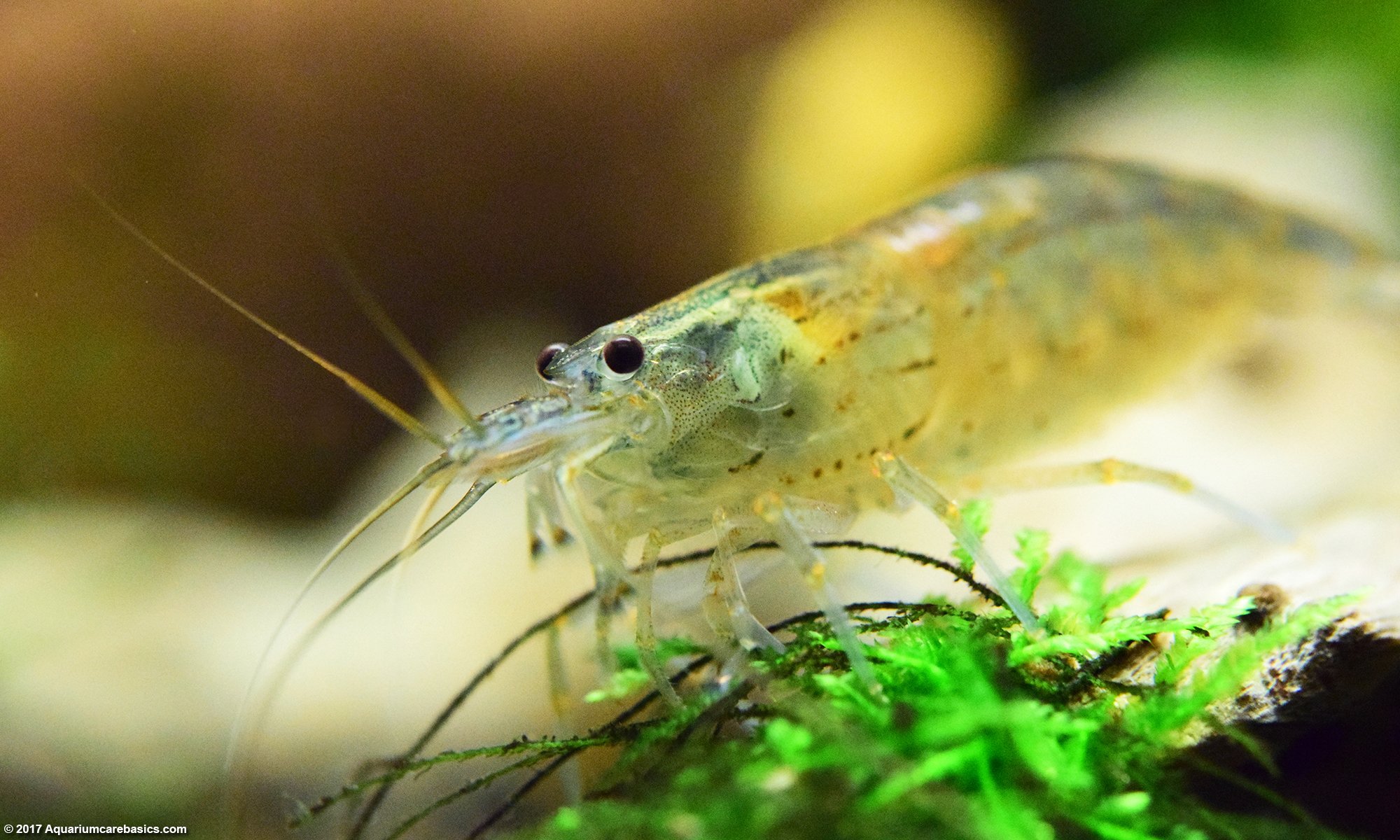This close-up photo captures a fascinating, semi-transparent insect with a long body, reminiscent of a shrimp or lobster. The insect's head is distinctly green, and it has two protruding, black googly eyes and green antennae. Its mouth or beak extends far in front and is adorned with tendrils or spikes. The bug's color palette features shades of green and yellow, with a hint of gray, giving it a somewhat clear appearance. It stands on thin legs atop a green leafy plant. The blurred background consists of earthy tones, including brown and lighter brown, with a yellow spot. There is a small text in the lower left-hand corner, reading "copyright 2017, aquarium, airbasics.com," suggesting it may be an underwater image.